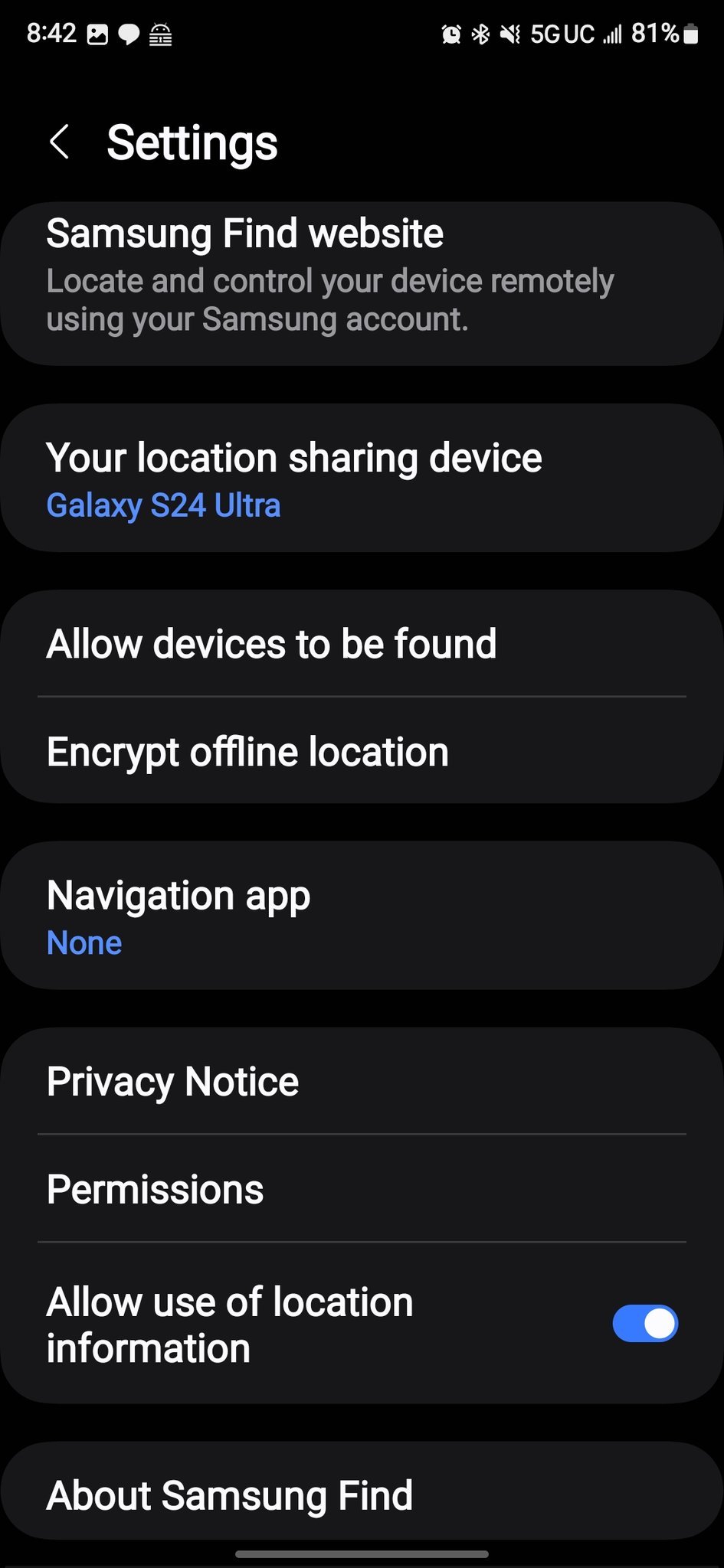This is a detailed caption for the image:

A screenshot of a settings page on a Galaxy S24 Ultra device, prominently labeled with "Settings" in white lettering against a black background. At the top left corner, the number "842" is displayed. The page shows a 5G UC connection with 81% battery remaining. The main section highlights "Samsung Find" and provides the description: "Locate and control your device remotely using your Samsung account." Below this, it indicates the currently shared device, "Galaxy S24 Ultra," and an option to "Allow devices to be found." 

There is an inactive option marked as "Inert offline location" and another unchosen option for a "Navigation app," listed as "None." A privacy notice mentions "Permissions" and prompts users to "Allow use of location information," with a blue and white toggle button on the right signifying that this setting is activated. 

At the bottom of the page, clickable options include "About Samsung Find." The text "Galaxy S24 Ultra" and "None" are featured in bright blue, while all other text is presented in white, providing a clear contrast against the black background.